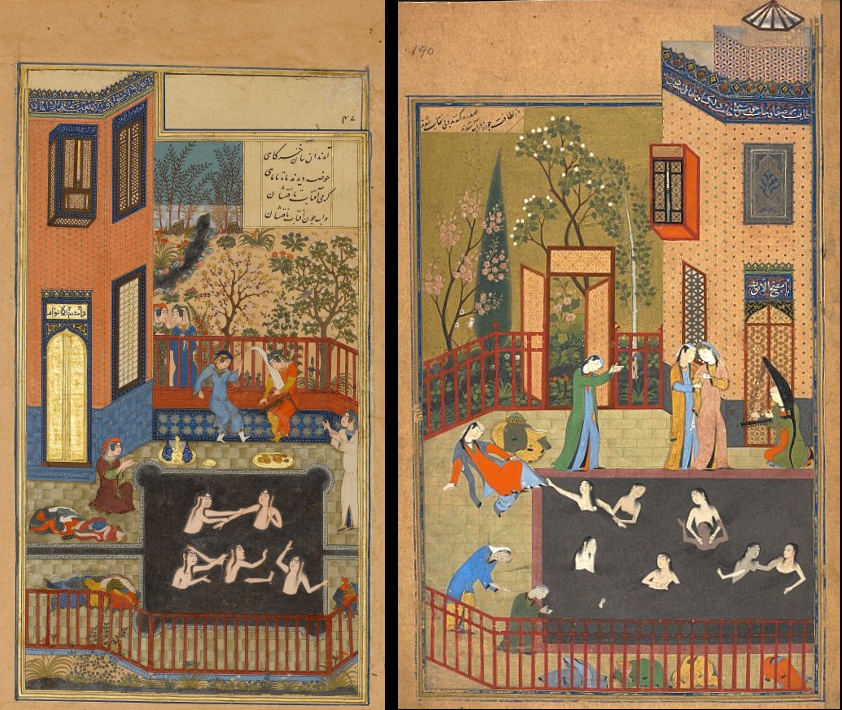This detailed illustration appears to be a diptych, possibly a Japanese or Chinese drawing, consisting of two interconnected scenes separated by a vertical black line. Both panels depict urban courtyard settings with bustling activity around swimming pools. 

On the left panel, a courtyard features a building with distinct blue and red brick patterns, adorned with three windows and a doorway. In front of the building, a garden blooms just beyond the pool's dark, almost black water. Within this pool, unclothed figures interact, possibly washing each other, with one holding the hands of another. Surrounding the pool, people sit on benches and engage in various activities, all framed by a red fence.

The right panel mirrors the left with a similar courtyard setup. Here, a cream and brown building with uniquely shaped windows stands, encircled by people clothed in multicolored outfits of green, yellow, orange, and blue. The pool, dark in color like the first, is filled with swimmers who touch and interact at the water's edge. More people stand, talk, and lounge around this area, framed by a garden and another tall building with ornate windows and architectural detailing.

Both scenes depict a lively, residential community environment rich in architectural detail and social interaction, where people of various ages gather around the central feature of the pools.